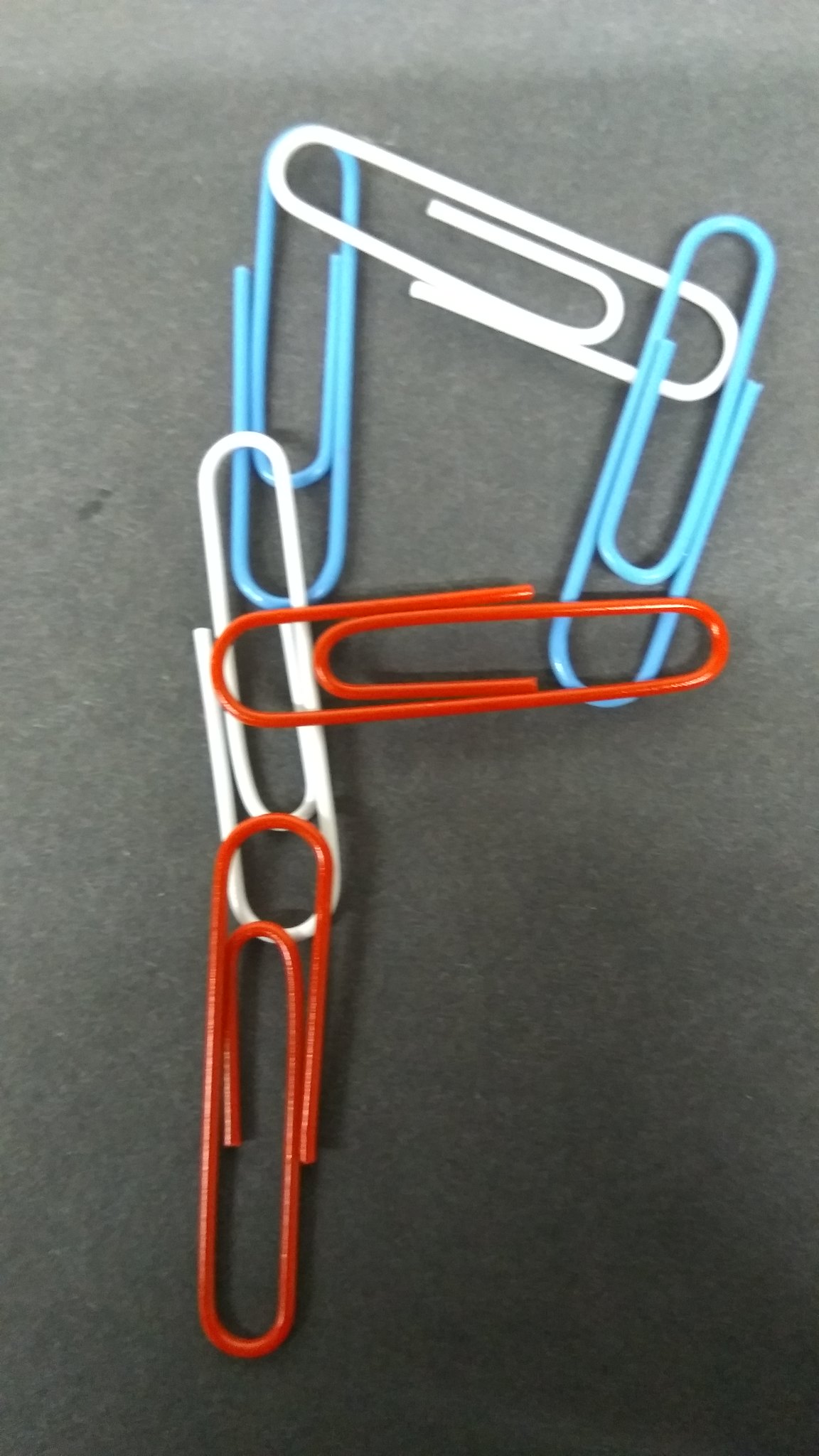The image features a gradient gray background that transitions from a deep charcoal gray at the bottom to a very light gray at the top. Centered in the image are six thin, shiny metal paperclips arranged to form the shape of the letter "P." The vertical line of the "P" starts at the bottom with a red paperclip, followed by a white paperclip in the middle, and a blue paperclip at the top. Extending to the right from the top of the blue paperclip is another white paperclip. Attached to the end of the white paperclip and curving downwards to form the rounded part of the "P" is a blue paperclip, which then connects to a red paperclip that curves back towards the left. The paperclips are in pairs of two red, two white, and two blue, and each is characteristically rounded and crafted from thin metal.